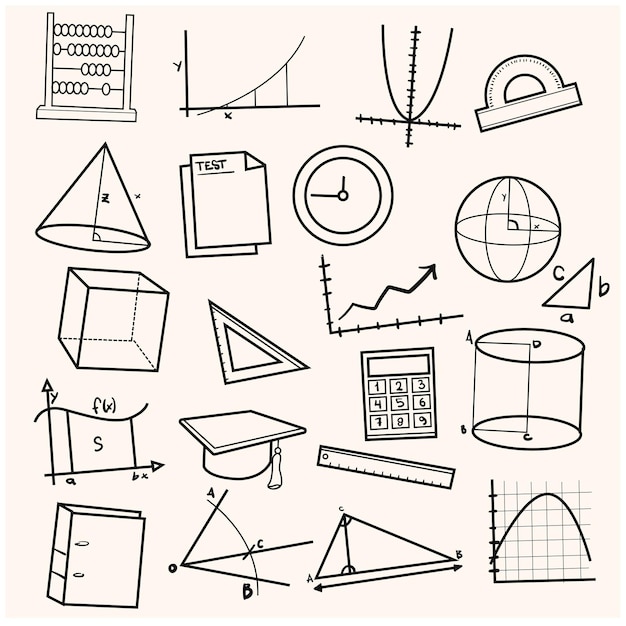A detailed black-and-white hand-drawn illustration depicts an assortment of mathematical and educational objects arranged in a grid with five rows and four columns against an off-white background. Starting from the top left, the first row features an abacus, followed by a graph with an upward slope, a parabola-shaped graph, and a measuring instrument with a flat edge and a circular end. The second row includes a cone, a pair of test papers (one with a dog-eared corner labeled "test"), a clock showing 11:45, and a spherical object with internal structures. The third row showcases a square box, a mathematic ruler, a 90-degree angle with an arrow, and a triangle marked with letters "CAB." The fourth row contains a calculator, a cylinder, a squiggly and straight-line pattern, and a graduation cap with a tassel. The final row features a ruler, a book, a series of algebraic problems, and a graph depicting a line that rises and falls. These intricately detailed images convey a realistic appearance, presenting a comprehensive assortment of school-related items and mathematical tools.